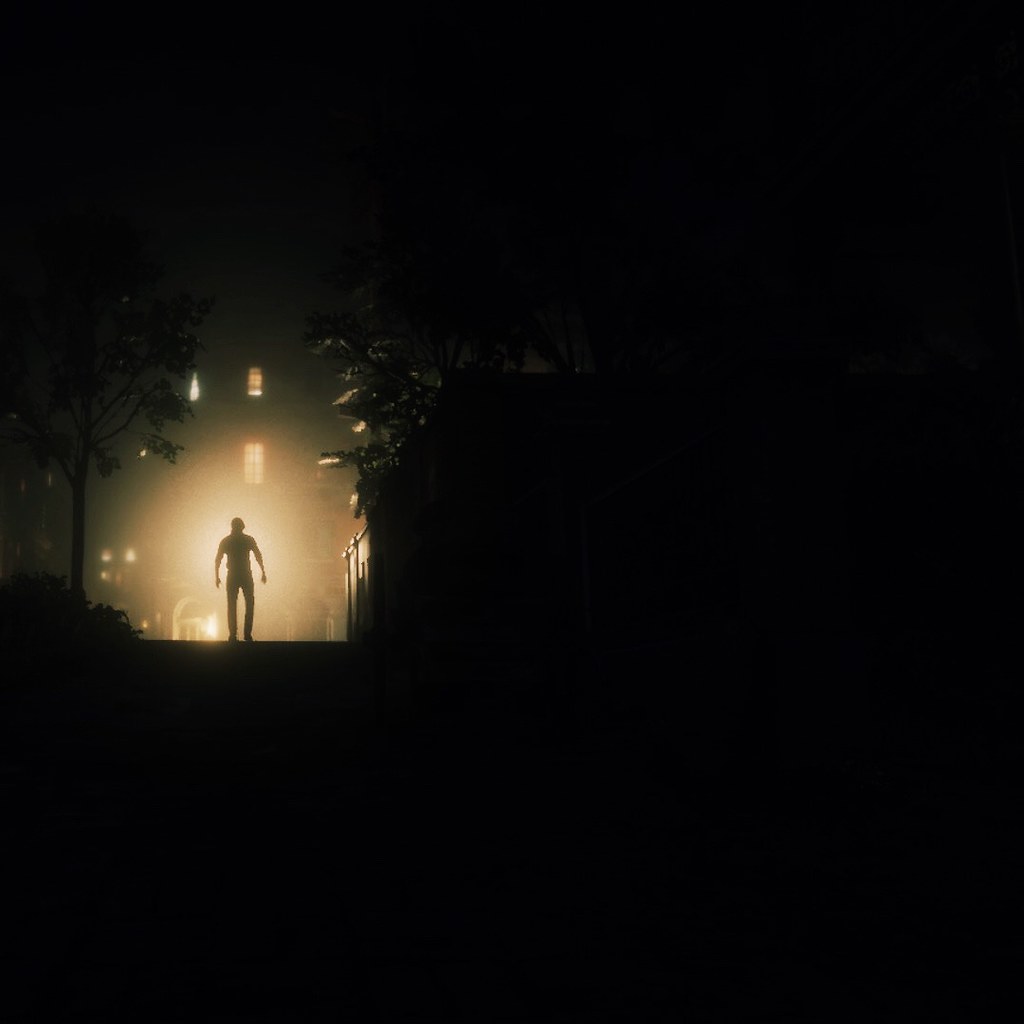The photograph exudes a creepy, horror movie aesthetic with an overwhelmingly black backdrop that engulfs most of the image. The bottom right, top right, and bottom left corners are completely shrouded in darkness, offering almost no visible details. Prominently in the center-left portion of the image, a bright yellow light illuminates the scene, casting an eerie glow. The light exposes a partial view of a building with several windows, some of which emit light. There are also street lamps and tree foliage subtly visible around the periphery. Central to the image, a silhouette of a man stands tensely with his arms slightly extended at his sides, creating a sense of foreboding. The light source behind him produces a dramatic sunburst effect, accentuating the spectral atmosphere. The overall scene is both mysterious and unsettling, dominated by pitch-black shadows and sporadic illuminated elements.